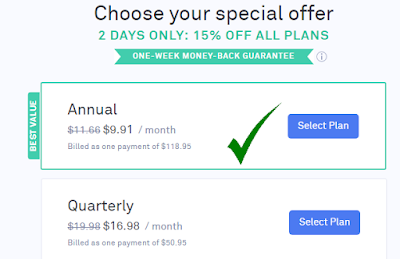The image features a promotional page for a subscription service with a compelling call to action at the top. In bold black text, the headline reads, "Choose Your Special Offer," followed by the subheading "Two Days Only: 15% off All Plans" in vibrant green. This limited-time offer also includes a "one-week money-back guarantee," ensuring customer satisfaction.

The promotional content is divided into two distinct subscription options: Annual and Quarterly. 

Under the Annual option, a green box prominently labeled "Best Value" with a large green checkmark grabs attention. Initially priced at $11.66 per month, this rate has been discounted and now shows a reduced price of $9.91 per month, clearly marked with a gray arrow. The total annual cost is $118.95, billed in a single payment. A blue "Select Plan" button below encourages immediate action.

The Quarterly option lists its original price as $19.98 per month, which is now reduced to $16.98 per month. This plan is billed quarterly at a total of $50.95. Like the annual option, it also features a blue "Select Plan" button.

The page design uses a predominantly white background with black text for readability, complemented by occasional splashes of vivid colors such as green and blue to highlight important details and make the deal visually appealing. The overall layout ensures clarity and directs attention to the key components of the offer.